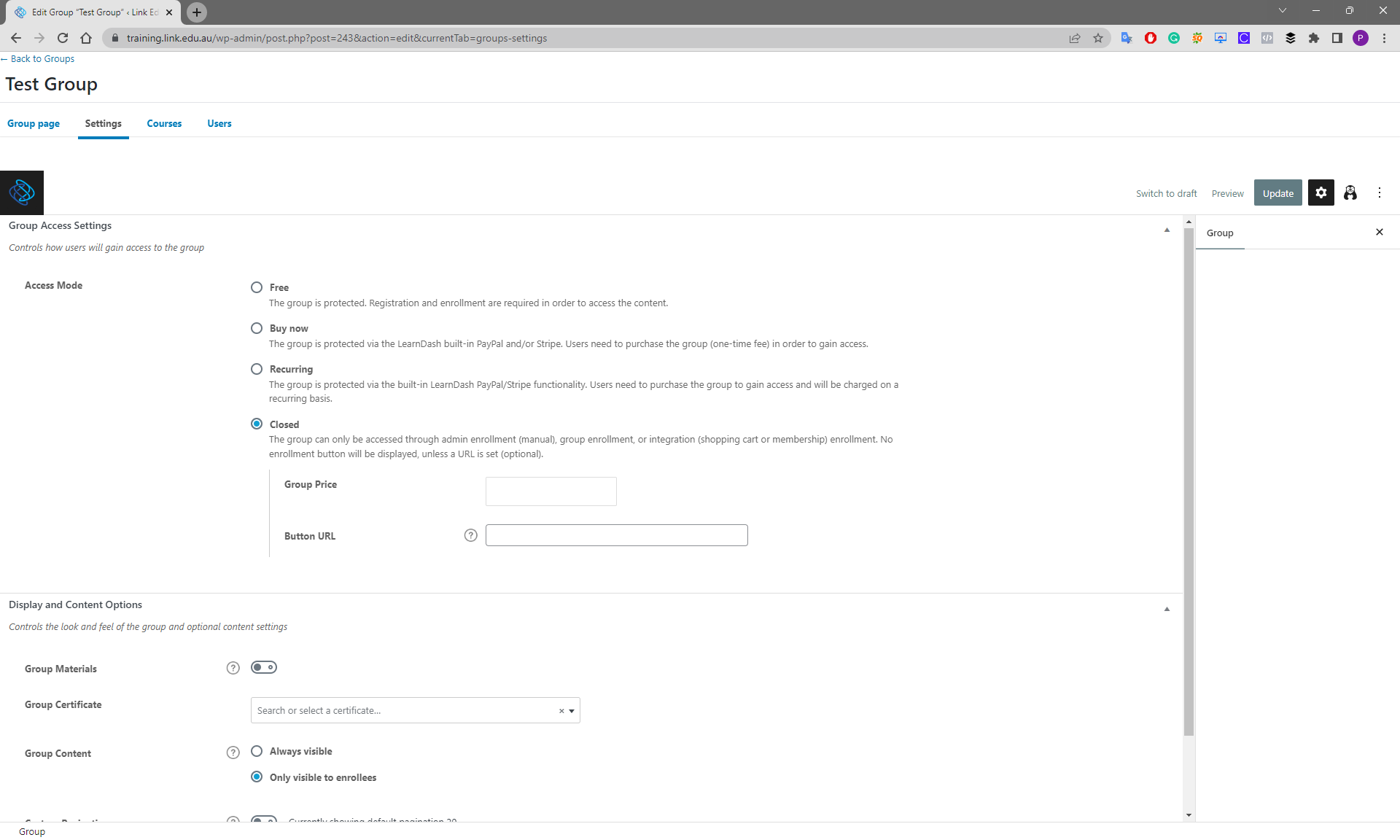Screenshot of a desktop web browser with a single tab open. The URL in the address bar, which appears to be from an Australian domain (.com.au), is not clearly legible. The website has a minimalistic design, characterized by a white background and black text. At the top, the headline reads "Test Group." There are several navigation tabs labeled: "Group," "Page," "Settings," "Course," "Courses," and "Users." The "Settings" tab is currently active, displaying various configuration options.

Under "Group Access Settings," the "Access Mode" section presents four options: "Free," "Buy Now," "Recurring," and "Closed," with the "Closed" option selected. Further down are sections for "Display and Content Options," featuring selections such as:
- "Group Materials"
- "Group Certificate"
- "Group Content"

Some options have question mark icons next to them, indicating the presence of additional information or tooltips.